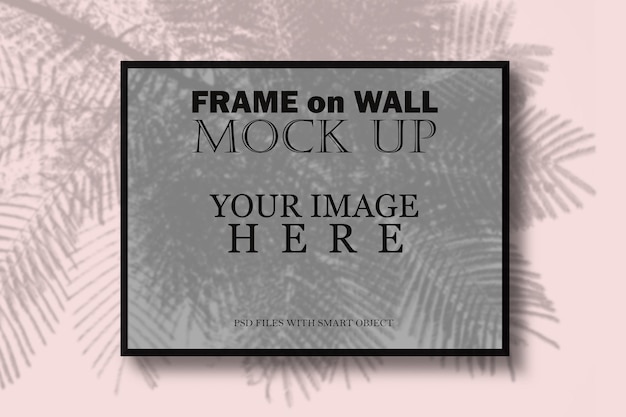The image features a light pink background adorned with a network of faded gray palm fronds extending in various directions. At the center, a black-framed rectangular space captures attention with a grayscale version of the palm frond pattern within it. The text in the frame is arranged in three distinct sections: at the top, in bold black font, it reads "Frame on Wall," with 'Frame' and 'Wall' capitalized. Beneath this, in a thinner and more stylized black font, it says "Mock-up." Below this, the text "Your Image Here" is printed in bold, with 'Here' spaced out as "H E R E." Finally, at the bottom, there's a smaller line of text that reads "PSD files with Smart Object." This detailed layout suggests the image serves as a template for displaying customizable content within the framed area.